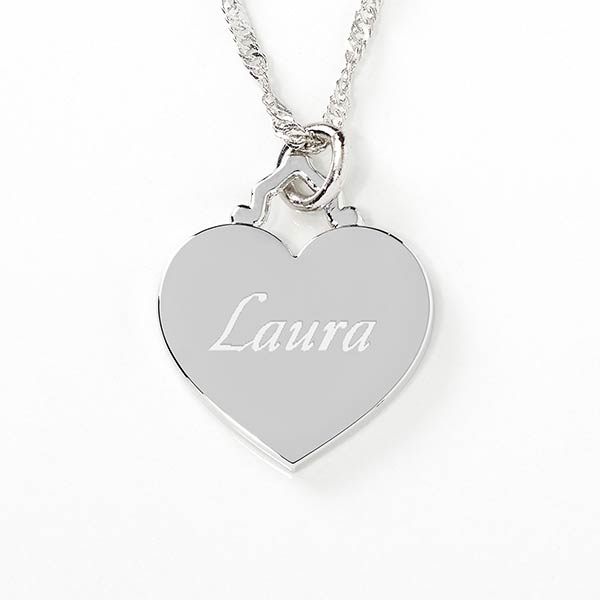This close-up photograph showcases a customized heart pendant necklace set against a plain white background. The pendant is crafted from shiny silver and features the name "Laura" engraved in a delicate, loose cursive type font, with each letter smoothly connected. The inscription is slightly lighter than the silver heart, creating a subtle contrast. The pendant is attached to a thin, delicate silver chain via a vertical pyramid-shaped piece and a round jump ring. The chain is partially visible, forming a V shape at the top of the image. This product photograph focuses exclusively on the pendant, highlighting its fine details and craftsmanship.